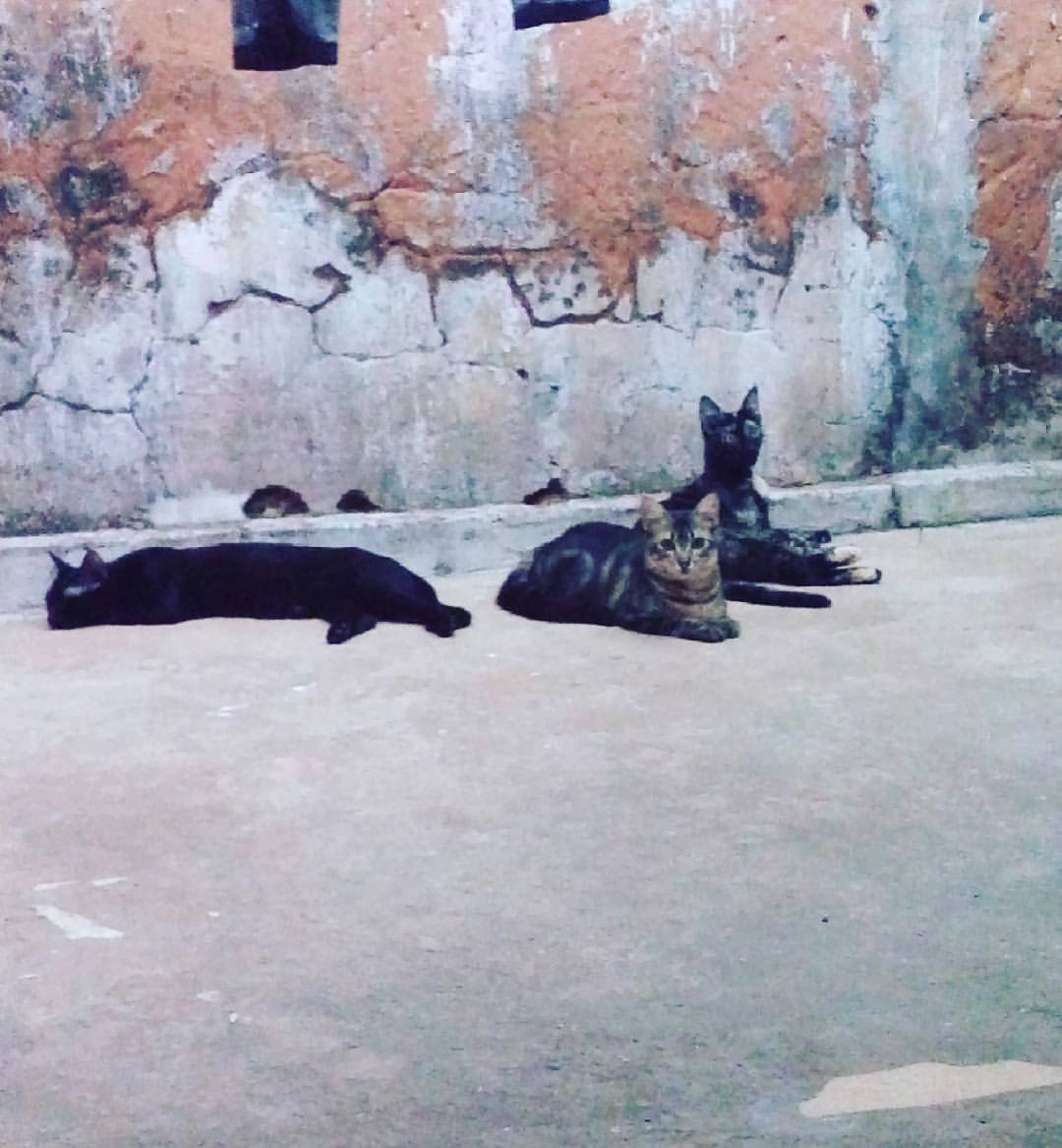In this detailed photographic image taken outdoors, three cats are lounging on a paved road alongside a deteriorating stone wall. The road's surface is gray and meets a similarly colored curb, leading up to the wall. This wall exhibits a distressed look, characterized by various hues such as light gray, orangish-brown, white, and clay, interspersed with darker and green spots, suggesting age and neglect. The wall displays extensive cracks, extending vertically and horizontally, with what appear to be hollowed-out, blackened windows towards the top.

In the foreground, near the curb, lie the three cats. The cat positioned on the left is entirely black, peacefully lying down. The cat in the center has a notable appearance—its body is predominantly black except for the chest and face areas, which feature a grayish-tan coloration with hints of beige and pink within its ears. This cat's posture is relaxed, seemingly observing the camera. To the right, the third cat, also black with gray specks or stripes, is slightly sitting up and peering off into the distance with alert brown paws. The scene captures a tranquil moment amidst an urban backdrop that tells a story of time and endurance.